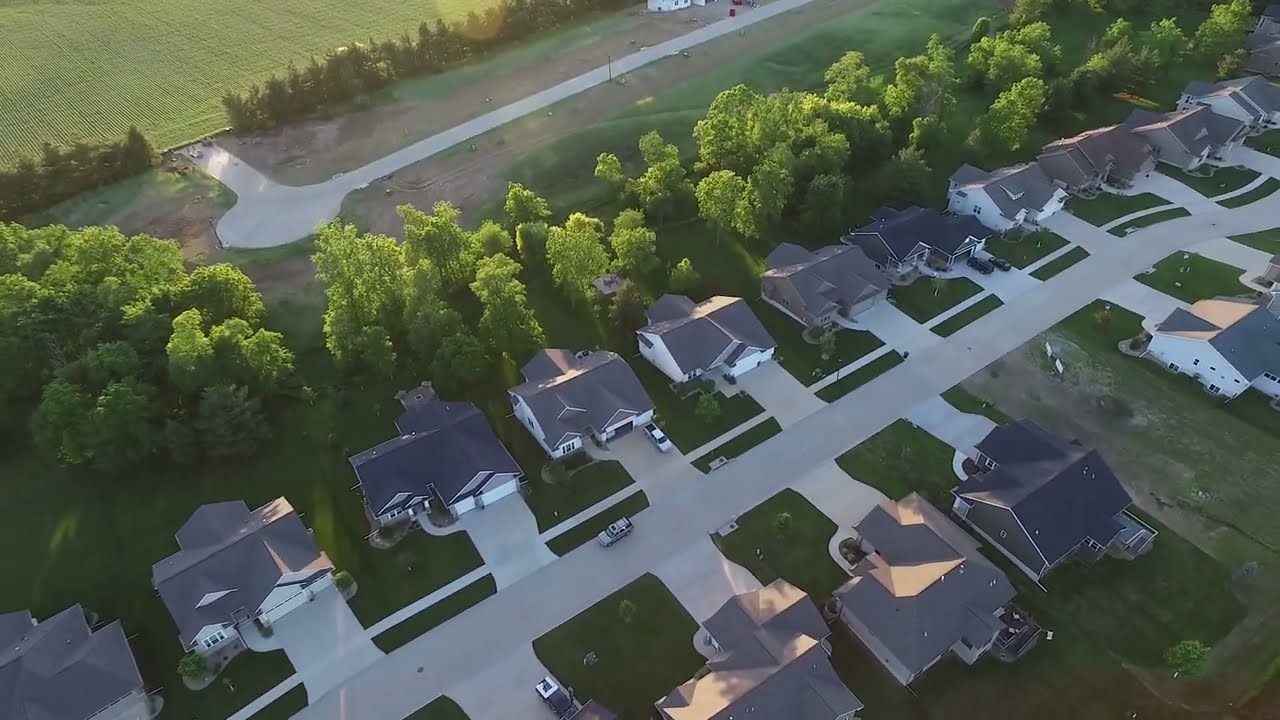The aerial view showcases a suburban neighborhood, characterized by its uniform houses lining both sides of a cement street. Each house, primarily featuring gray or dark gray roofs, comes equipped with double car garages and driveways, reflecting their three to five-bedroom size. The houses sport varied sidings in white, brown, tan, and darker shades of these colors. Neatly kept green lawns extend to a sidewalk that runs parallel to the street. Scattered cars in driveways and on the street complement the tranquil residential scene.

To the left side of the street, a row of lush, light-green trees forms a natural boundary, beyond which lies an expansive stretch of dark green grass leading to a farm-like area. In the distance, rows of crops hint at tilled farmland, and a white portion of a house peeks through this greener landscape. The sun bathes the entire scene, enhancing the vibrancy of the summer greenery. A dirt road and additional trees serve as further boundaries, encapsulating this peaceful subdivision.